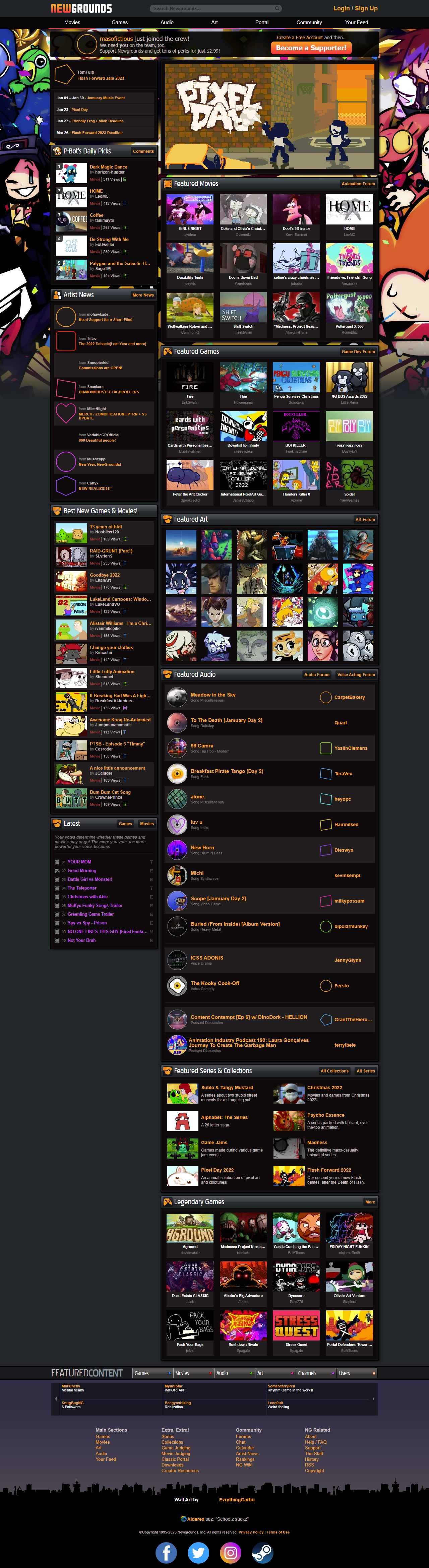This screenshot from the website Newgrounds highlights its vibrant and engaging interface. The image quality appears to be somewhat shrunken or reduced. At the top of the page, a black bar displays the site name "Newgrounds" with "new" in orange and "grounds" in white. To the right of the logo is a search bar, along with orange buttons for login and sign-up functions.

On the left side, there is colorful artwork featuring various characters, including a parrot and some human figures. Similarly, the right side also displays additional character artwork. Running down the left side of the page, there's a "Dailies Pick" section, showcasing a curated selection of games and movies. Below this is the "Latest" section, providing updates on newly added content.

The central part of the page prominently features a selection of games and movies in a "Featured" section. Finally, at the very bottom of the screenshot, there are social media icons for Facebook, Twitter, Instagram, and Steam, facilitating easy navigation to Newgrounds' respective social media pages.